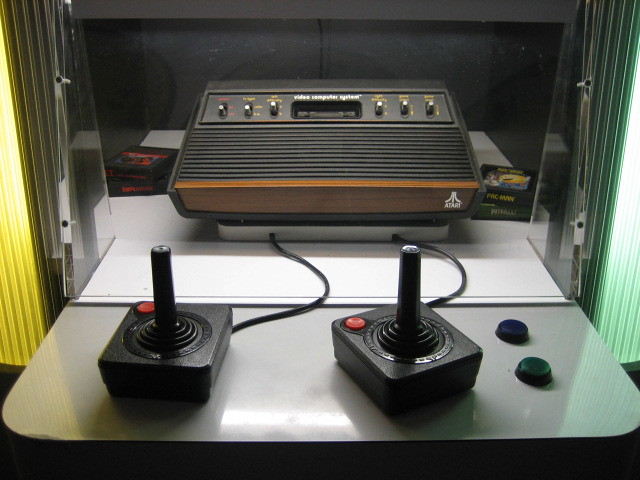The image showcases a classic Atari video game console from the 1980s, prominently displayed in a museum-like setting. The console is encased in a protective clear box, emphasizing its historical significance. It features a distinctive brown wood base with the "Atari" logo prominently displayed in white lettering. The top section of the console is adorned with an array of metallic buttons. Connected to the console are two handheld controllers, each equipped with a dynamic joystick that allows for multi-directional movement, along with a single red button located in one corner for gameplay interactions. These controllers are placed outside the clear case, inviting museum visitors to handle and experience them firsthand. Additionally, the display stand integrates two color-coded push buttons, one blue and one green, enhancing the interactive experience of the exhibit.